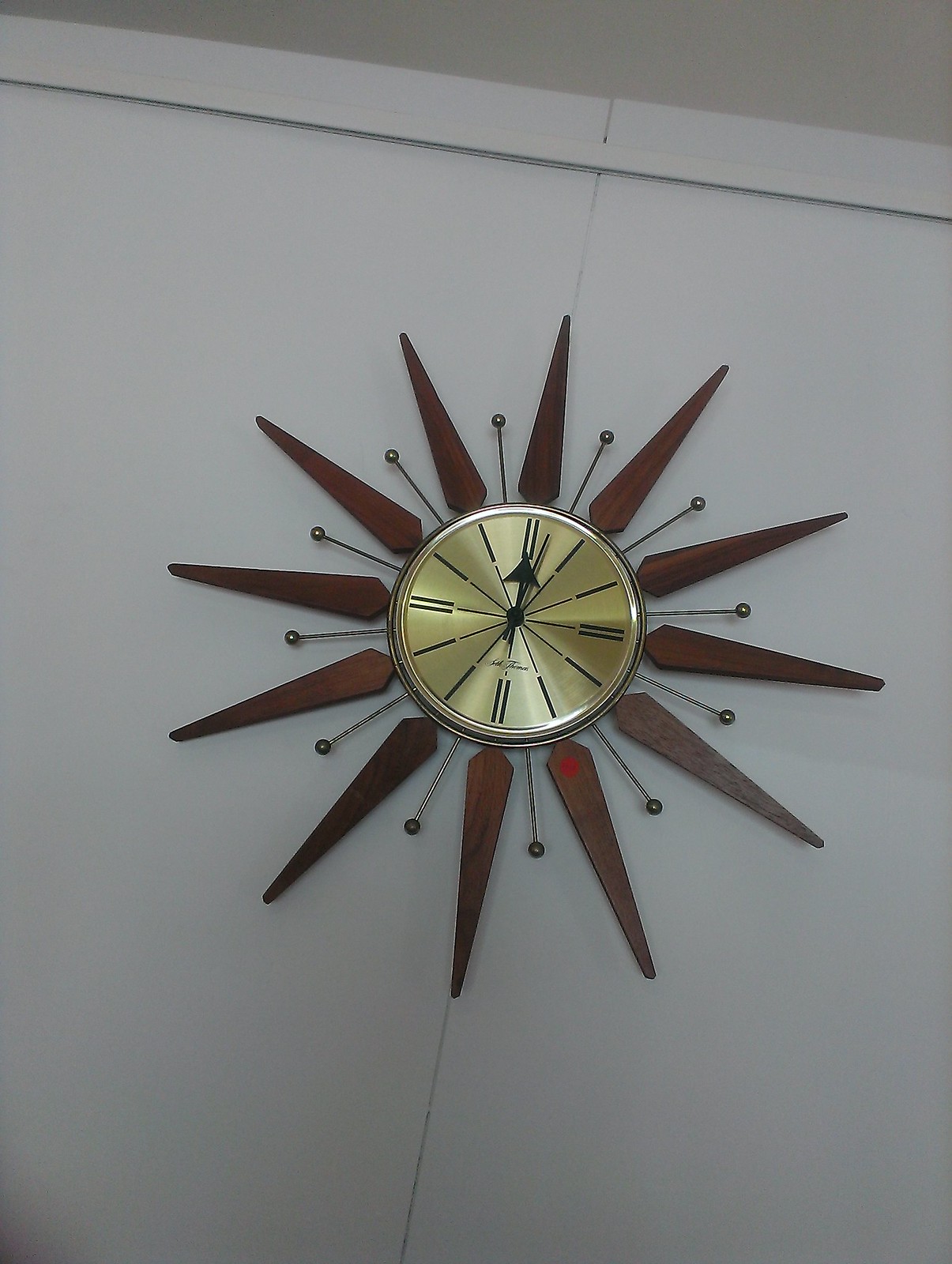The photograph features a striking mid-century modern wall clock hanging on a white wall. The clock displays a distinctive sunburst pattern crafted from wooden rays that extend outward. Each wooden ray is wide at its base near the clock face and tapers to a thin point, accentuating the sunburst effect. Nestled between these wooden rays are smaller metallic rays, adding an intricate detail to the overall design. The clock face is a glistening gold or brass color, with black Roman numerals at the 12, 3, 6, and 9 o'clock positions and simple black lines marking the other hours. The clock's frame is also golden, complementing the clock face. The hands of the clock are black, with thick and prominent minute and hour hands. The time reads a couple of minutes past 12. The photograph is taken from a slightly tilted angle, revealing that the wall is divided by a thin crack and features a molding at the top, both of which are the same white as the wall.